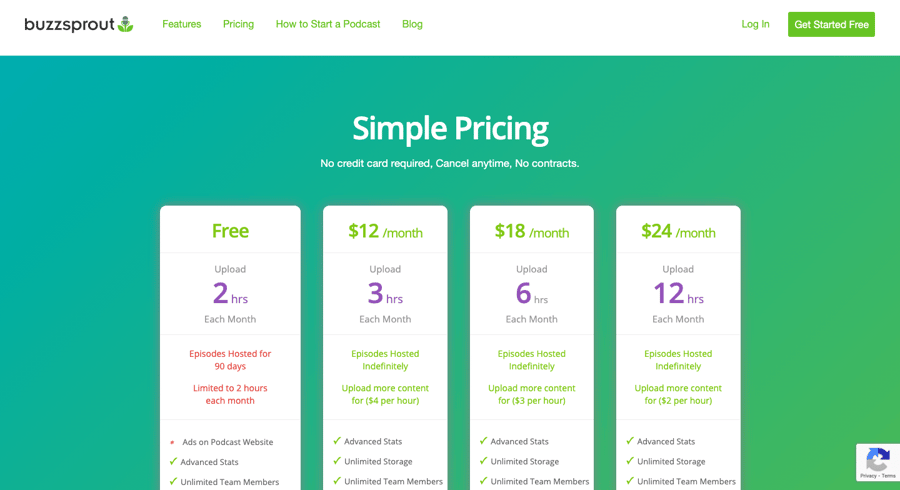In this image, we see a detailed screenshot from the Buzzsprout website. Buzzsprout, spelled B-U-Z-Z-S-P-R-O-U-T, offers an array of features and information designed to guide users on starting a podcast. The menu on the left side includes options like Features, Pricing, How to Start a Podcast, and Blog. On the right, there are buttons for Login and Get Started Free highlighted in red.

Prominently displayed in the center is a large aqua-colored section with the headline "Simple Pricing" in bold white letters. Beneath this, phrases like "No credit card required," "Cancel anytime," and "No contracts" emphasize the flexibility of their service plans.

The pricing details are organized into four tiers:

1. **Free Plan**
   - **Upload Limit:** 2 hours each month
   - **Hosting Duration:** Episodes hosted for 90 days
   - **Additional Features:** Ads on podcast website (not included), advanced stats (included), unlimited team members (included)

2. **$12/month Plan**
   - **Upload Limit:** 3 hours each month
   - **Hosting Duration:** Episodes hosted indefinitely
   - **Additional Upload Cost:** $4 per additional hour
   - **Additional Features:** Advanced stats, unlimited storage, and unlimited team members (all included)

3. **$18/month Plan**
   - **Upload Limit:** 6 hours each month
   - **Hosting Duration:** Episodes hosted indefinitely
   - **Additional Upload Cost:** $3 per additional hour
   - **Additional Features:** Advanced stats, unlimited storage, and unlimited team members (all included)

4. **$24/month Plan**
   - **Upload Limit:** 12 hours each month
   - **Hosting Duration:** Episodes hosted indefinitely
   - **Additional Upload Cost:** $2 per additional hour
   - **Additional Features:** Advanced stats, unlimited storage, and unlimited team members (all included)

Overall, the screenshot provides a comprehensive view of Buzzsprout's user-friendly and tiered pricing structure, with various features tailored to meet the needs of different podcasters.